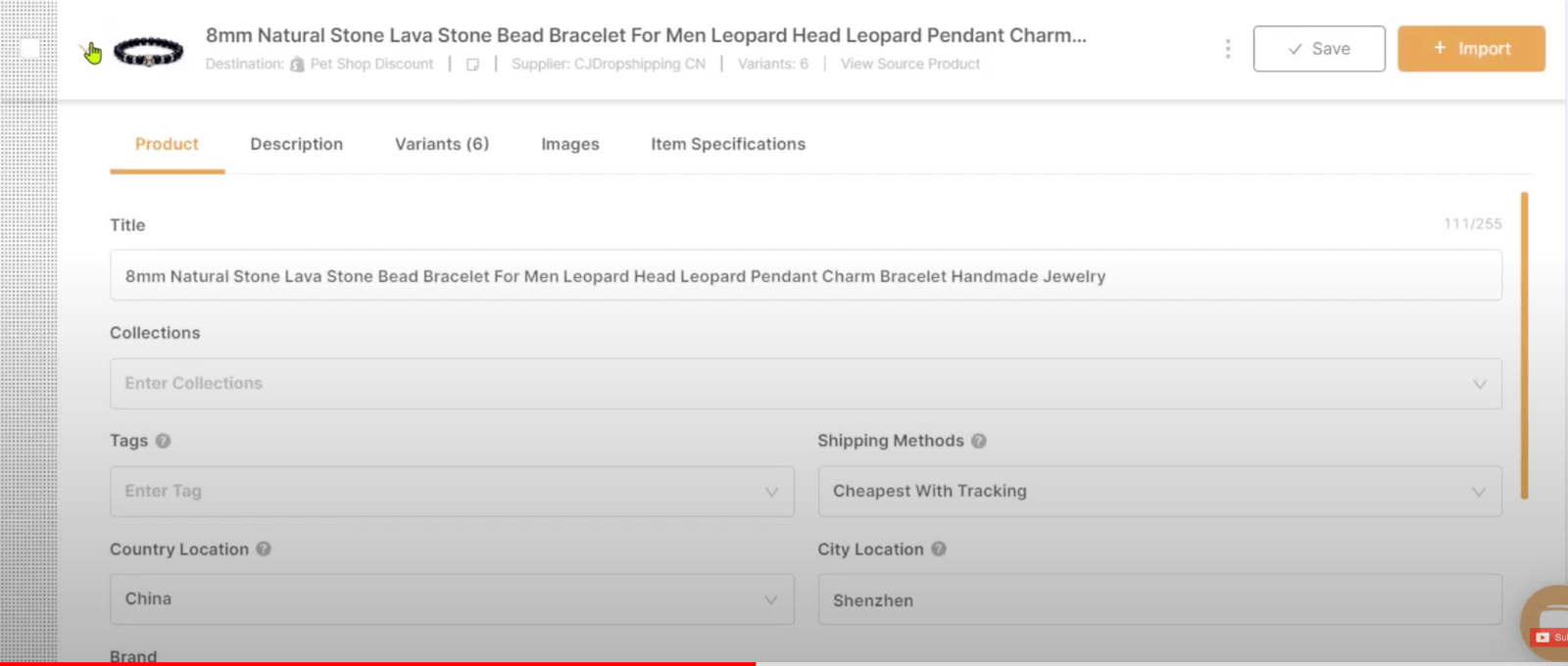This image is a screenshot of a product listing page on a website, featuring a predominantly white background. On the left-hand side, a vertical gray bar with black text displays the product's title: "8mm Natural Stone Lava Stone Bead Bracelet for Men Leopard Head Leopard Pendant Charm." Adjacent to this bar is a small image of the bracelet itself, which consists of black beads and is described disdainfully as "ugly." To the right of the bracelet's image, gray text details additional information: "Destination, Pet Shop Discount, Supplier, CJ Drop Shipping CN, Variant 6, View Source Product."

On the far right of the screenshot, there are two buttons: a white "Save" button and a green "Import" button. Below these buttons is a menu with several tabs: Product, Description, Variants (6), Images, and Item Specifications. The "Product" tab is currently selected.

Under the selected tab, the page shows a "Title" field with the pre-filled text: "8mm Natural Stone Lava Stone Bead Bracelet for Men Leopard Head Leopard Pendant Charm Bracelet Handmade Jewelry." Following this are sections labeled "Collections" and "Tags," both of which have empty input boxes. Lastly, the "Shipping Methods" section indicates the option selected as "Cheapest with Tracking."